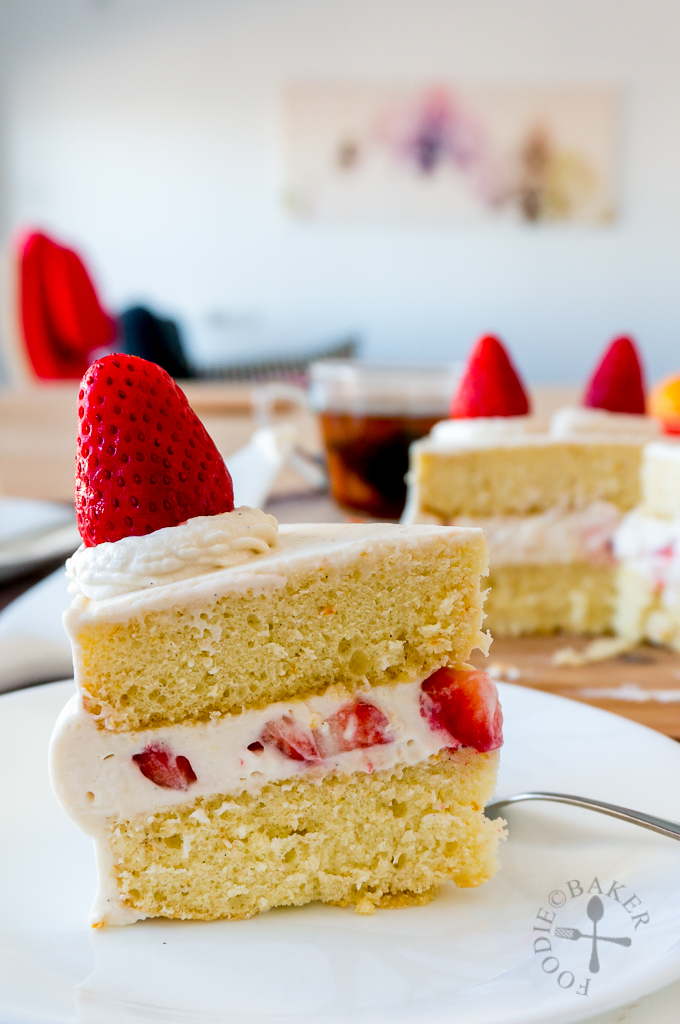This detailed close-up photograph showcases a delectable piece of strawberry shortcake on a white plate, accompanied by a piece of silverware, presumably a fork. The cake features two yellow layers of soft cake, with a central layer of white frosting embedded with juicy, cut strawberries. Crowned with a large, perfectly ripe strawberry, pointed end up, it looks incredibly appetizing. Blurred in the background are additional pieces of similar cake and some kind of drink, all set on a wooden table. Also present in the out-of-focus background is a piece of art hanging on the wall. The photograph includes a watermark in the lower right corner, showing the moniker "Foodie Baker" next to a crossed fork and spoon icon in gray, adding a subtle touch of professionalism. The overall presentation is immaculate and inviting, capturing the essence of a well-crafted dessert.